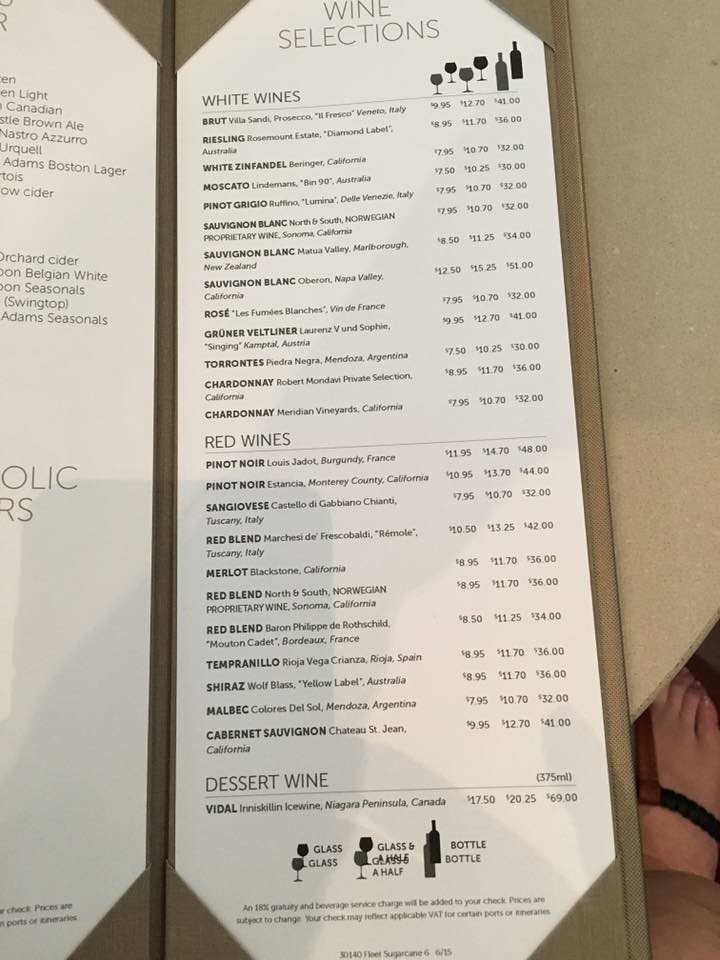This detailed image captures a long, narrow, vertically-oriented menu folder comprising two pages. The menu prominently features a wine selection, displayed on the right page, consisting of a white paper backdrop with dark ink. The heading "Wine Selection" crowns the page, followed by a section for "White Wines." This section visually distinguishes itself with artistic images of two bottles and four wine glasses to the right side of the text. Within this part, approximately 13 different wine varieties are listed, including notable mentions such as Pinot Grigio, Rosé, and two types of Chardonnay. Each wine is presented with three prices: for a glass, a small carafe, and a full bottle. For instance, the Riesling, which is second from the top, is priced at $8.95 per glass, $11.70 for a carafe, and $36 for a bottle.

Below the white wines, the menu follows a similar layout for red wines, listing options like Red Blend, Merlot, and multiple entries for Pinot Noir. At the very bottom of this side, there is a distinct "Dessert Wine" section that features a single offering, Vidal. It is noteworthy that the mid-range price in this section denotes a glass-and-a-half serving rather than a carafe.

On the opposite left page, partially visible, is what appears to be a beer list. Only a quarter of this page is discernible, showing words such as Brown Ale, Canadian, Light, Adams, Boston, and Lager, suggesting a variety of beers offered.

The menu is skillfully designed to provide clear and organized choices for the patrons, making their dining and drinking selection experience pleasant and intuitive.